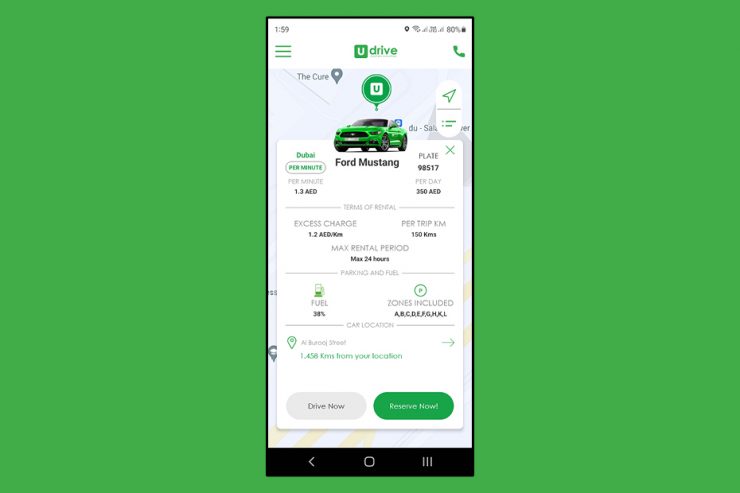The image is a detailed screenshot taken from a mobile device, showcased against a green background. The screenshot displays essential information such as the time (1:59), Wi-Fi connectivity, carrier signal strength, battery life at 80%, and that location services are enabled. At the top left of the screenshot, three green lines are visible, indicating a menu icon. Next to it is a green square with a white "U" on it, representing the "Udrive" app. 

In the upper section of the app display, there is a green handset icon for making calls, followed by a green Ford Mustang image. The app indicates car rental details, stating the rate for Dubai at 1.3 AED per minute and listing the vehicle's license plate as N8517 (or 98517). The daily rental rate is 350 AED, with an excess charge of 1.2 AED per kilometer. The car's fuel level is shown to be at 38%. Additionally, the maximum rental period is specified as 24 hours, with a limit of 150 kilometers per trip.